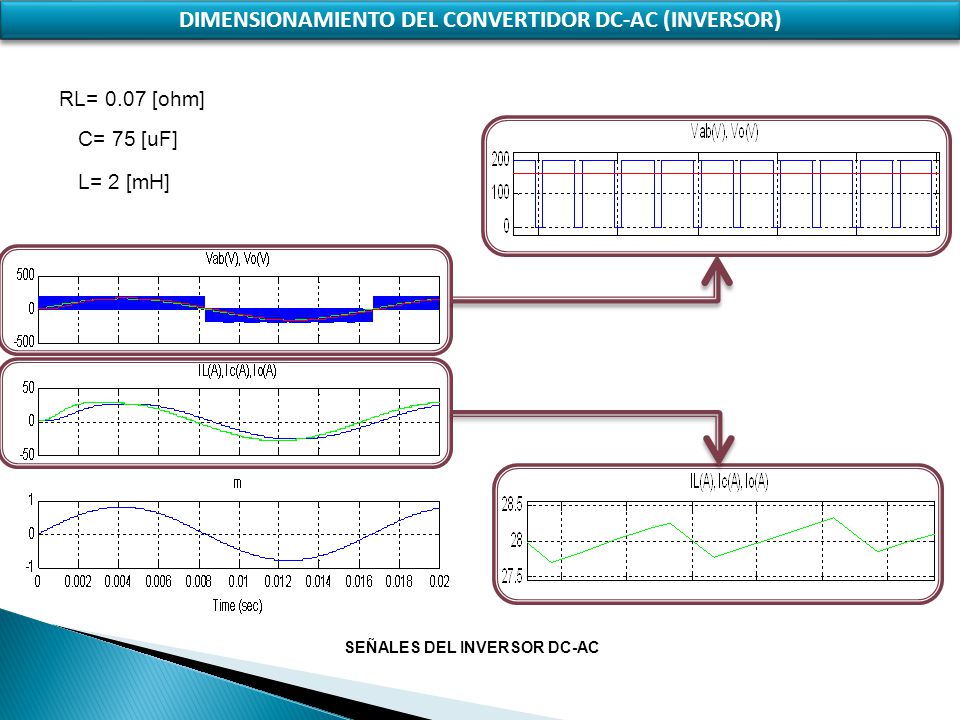This detailed infographic, titled "Dimensionamiento Del Convertidor DC-AC (Inversor)" in a thin blue band at the top, presents several interconnected graphs and equations essential for understanding DC-AC inversion. Below the title, on the left-hand side, there are three labeled variables: RL equals 0.07 (Ω), C equals 75 (µF), and L equals 2 (mH). To the right of these equations, a series of rectangular boxes contain graph charts connected by directional arrows. 

The first rectangular box on the left, containing a chart with a line pointing upwards, connects to another rectangular box on the right. Beneath it, another boxed chart directs an arrow downward to a third rectangular box below, which features a green line chart. Adjacent to these, a final chart in the bottom left corner displays a blue waveform graph, with its horizontal axis labeled "Time (s)" and its vertical axis marked from -1 to 1.

At the very bottom left of the graphic, there is a wedge shaped color gradient progressing from blue to black to light gray. To the right of this color gradient, the words "Señales Del Inversor DC/AC" are prominently displayed, detailing the context and purpose of the infographics and charts depicted.